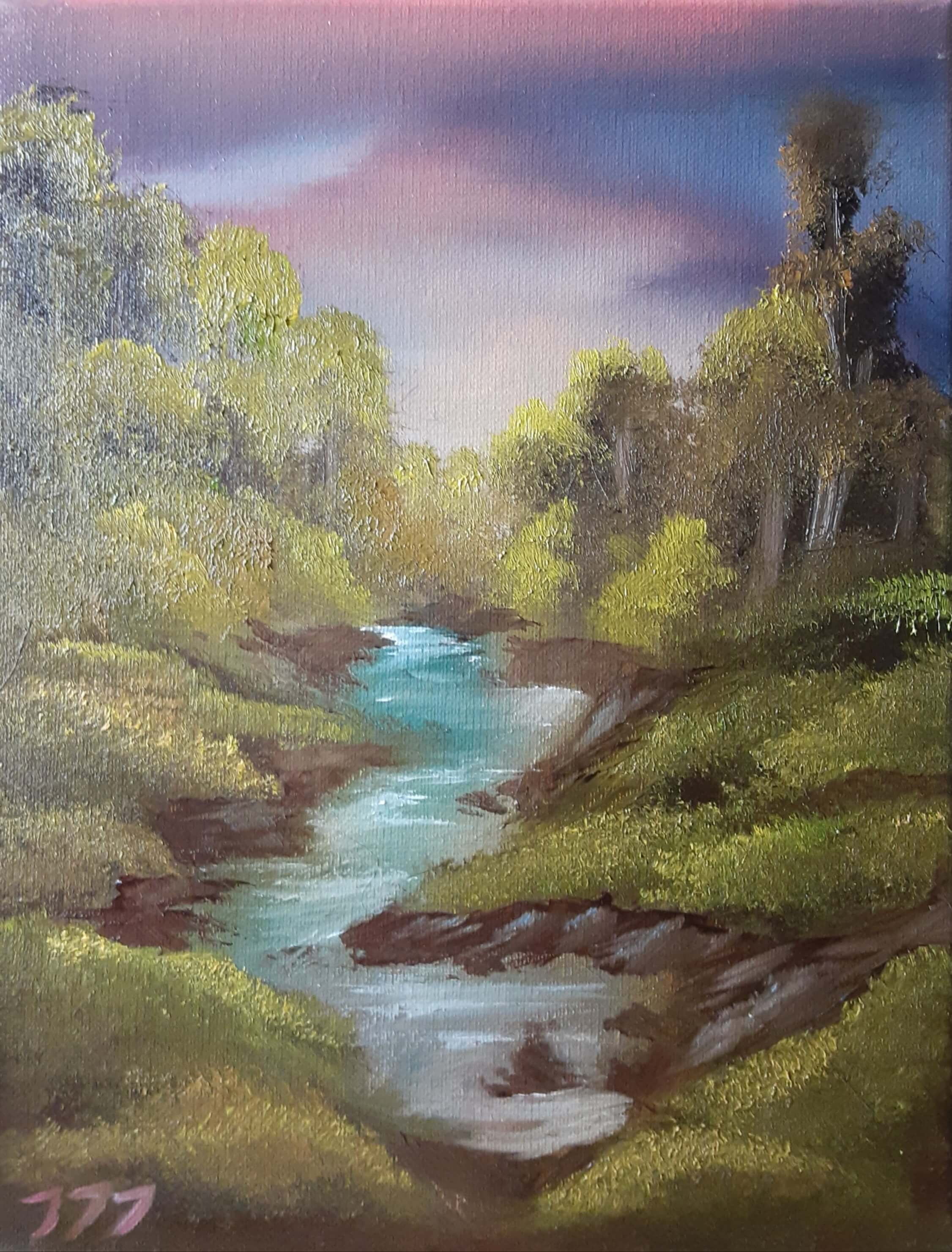This painting portrays a serene river landscape, winding its way through verdant shores. On both sides of the river, there are lush green trees and grasses, suggesting a thriving, deciduous forest. The river itself flows with greenish water, accented by white-painted ripples that convey motion. Along the banks, the ground slopes gently upward, adorned with grasses and shrubs, forming natural, landscaped shelves. Brown mugs are positioned near the riverbank, adding a rustic touch to the scene.

Above, the sky transitions from a deep blue at the top to a purplish pink near the horizon, indicative of a sunset scene. The clouds blend pink and gray hues, enhancing the atmosphere. In the bottom left corner of the painting, the artist has included the number '777' in pink, resembling a signature. The overall composition captures a tranquil, almost idyllic moment in nature, bathed in the soft, colorful light of an evening sky.